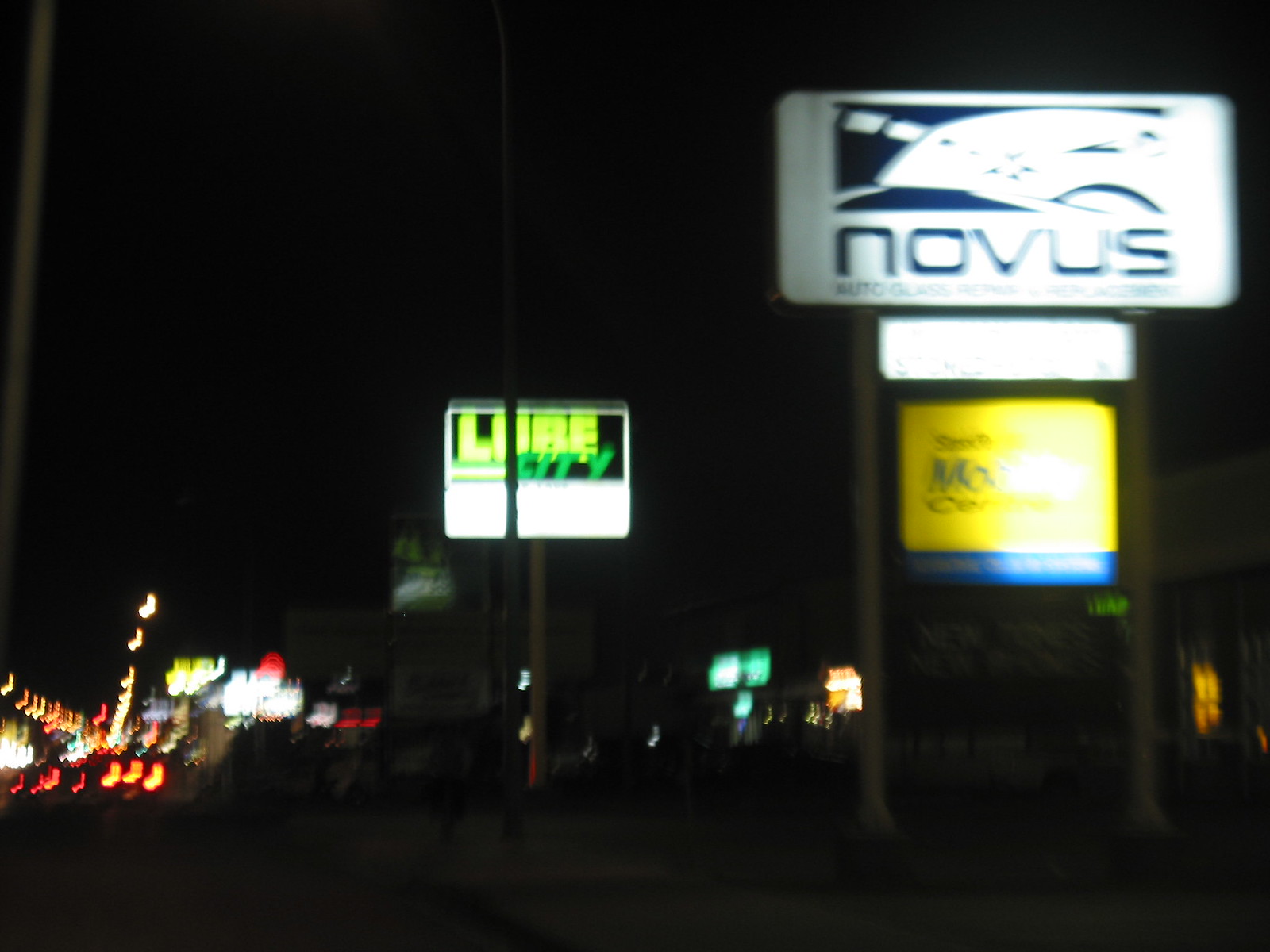The image depicts a lively cityscape at nighttime, with a black sky serving as a backdrop for a series of illuminated shop signs. The most prominent sign is on the right-hand side, displaying the word "Novus." Above the text, there is a white shape on a bluish background, though its exact form isn't clear. Below this, there are two more signs: one white and illegible, and another yellow sign with an unreadable inscription and a small blue section at its base.

To the left of the "Novus" sign, a bright yellow sign with "Lure" written in green can be seen, mounted on a white pole. Beneath this, there appears to be a white spot or light source. 

In the bottom left of the image, the scene extends to include streetlights, suggesting other shops and the taillights of passing cars. Additional shop fronts with illuminated signage are also visible in the bottom right corner, adding to the vibrancy and depth of the nighttime city setting. Despite these bright spots, much of the image remains cloaked in darkness, emphasizing the contrast between the illuminated signs and the night sky.